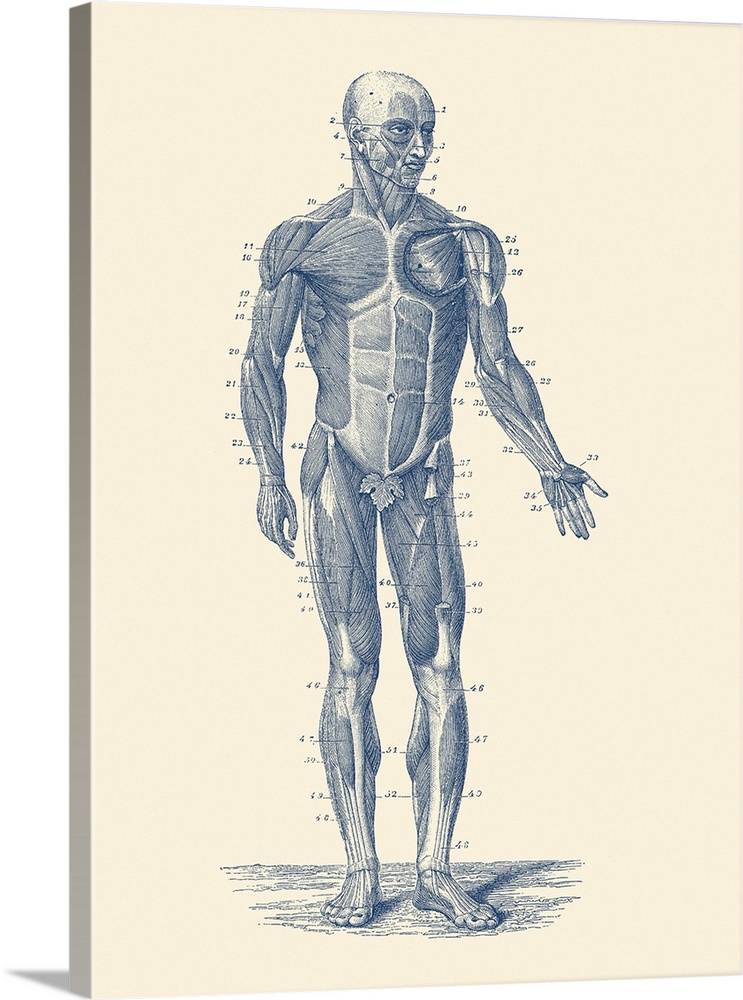This detailed anatomical diagram is sketched in black and white ink on a pale yellow, tan-colored background that resembles canvas. The human figure in the drawing is hairless, showing all muscle groups in meticulous detail, each identified by numbers ranging from 2 to 49. Depicted in a slightly angled frontal view, the male figure stands with his head turned to the side, left arm partially outstretched, and right arm resting by his side. A leaf is illustrated over the genital area for modesty. Numerous tiny lines point from each muscle to its corresponding number. The image emphasizes the complexity of the muscular structure, with every muscle from head to toe distinctly labeled.